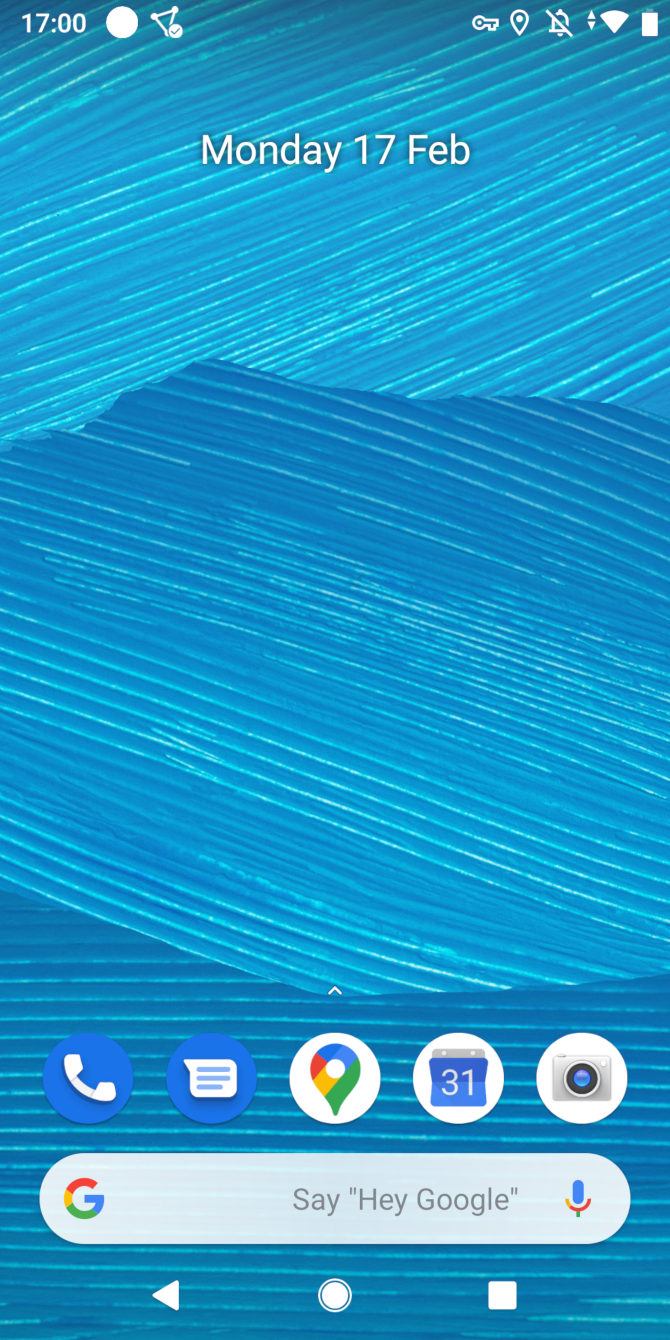Here is a detailed and cleaned-up caption for the image:

The image is a screenshot of a mobile phone's home screen. At the top, the status bar features various icons. From left to right, it shows the time "17:00" in a small white font, followed by a thin triangle made of lines, a sideways key icon, a location pin, and an outlined bell with a slash through it, indicating notifications are silenced. There is also an icon representing a windshield for WiFi service, and a vertical white battery bar.

Below the status bar, in the middle of the screen, a thin white font displays the date: "Monday, 17th Feb."

The wallpaper in the background consists of diagonal lines that shift in color. The pattern starts with light blue lines at the top leading to the left, transitions into darker blue in the middle going to the right, and ends with horizontal lines at the bottom.

At the bottom of the screen, there is a blue circle icon depicting the side view of a phone in white. Next to it, there is another blue circle with a white chat bubble icon. In the center of the bottom row of icons is the Google Maps app icon, resembling a stylized hot air balloon in blue, green, and red. To its right is a white circle with a calendar showing "31" and a grey, front-facing camera icon within a white circle.

Below the icons, there is a search bar that says "Say 'Hey Google'" in parentheses. To the right of the search bar is a microphone icon in blue and red.